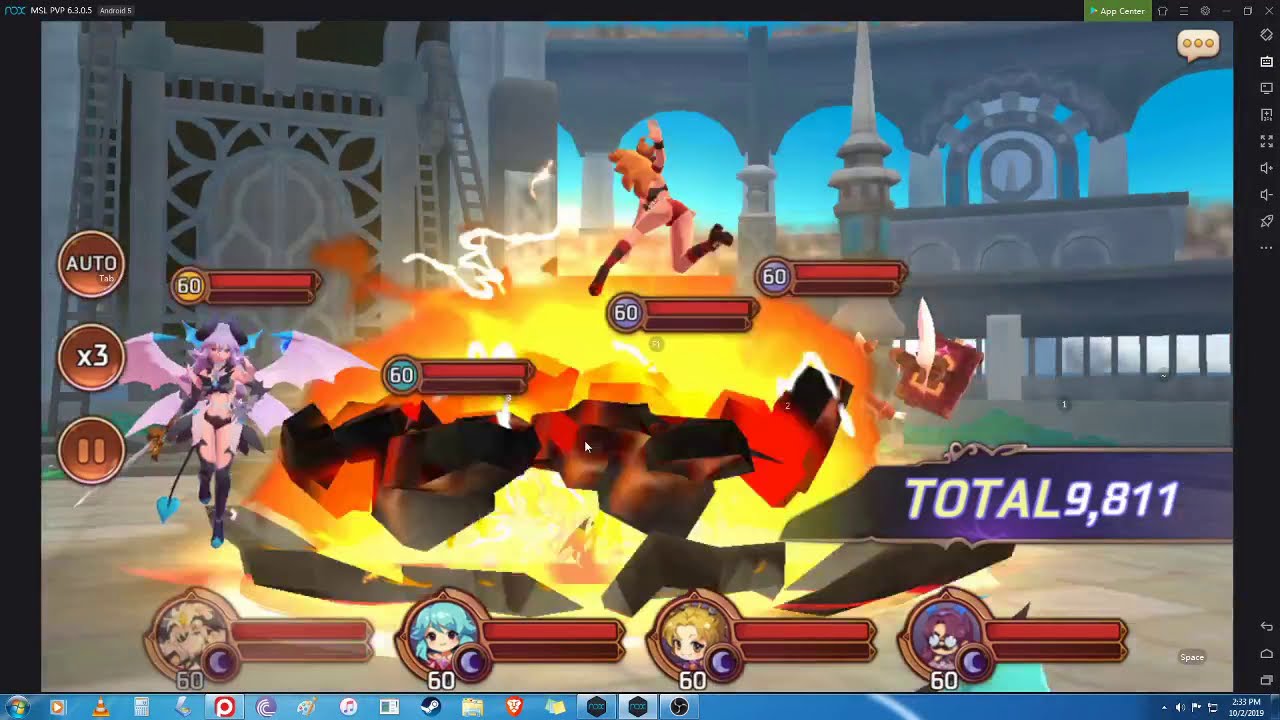This is a detailed screenshot of a vibrant and animated video game being played on a Windows computer, as evidenced by the visible Windows taskbar at the bottom of the screen. The scene is set in a coliseum with a bright turquoise sky and a backdrop of gray bridges and columns. The primary action features a dynamic fight sequence involving four anime-styled female characters, each with distinct appearances and health bars indicating '60' in white. One character, who appears to be a superhero with long purple hair and a mustache, is mid-jump above a fiery explosion of orange, yellow, and white. Another character with wings and a black two-piece outfit, knee-high socks or boots, has complex features including four pink wings with blue tips and a black tail ending in a white or blue spear. The other characters sport vibrant turquoise blue, gold, royal purple, and light yellow hair. The game's interface shows various character icons and a purple ribbon displaying a total score of 9,811 points. Additional indicators, such as an 'Android 5' label and an 'App Center' mention in the top corners, suggest the game could also be run on a tablet.